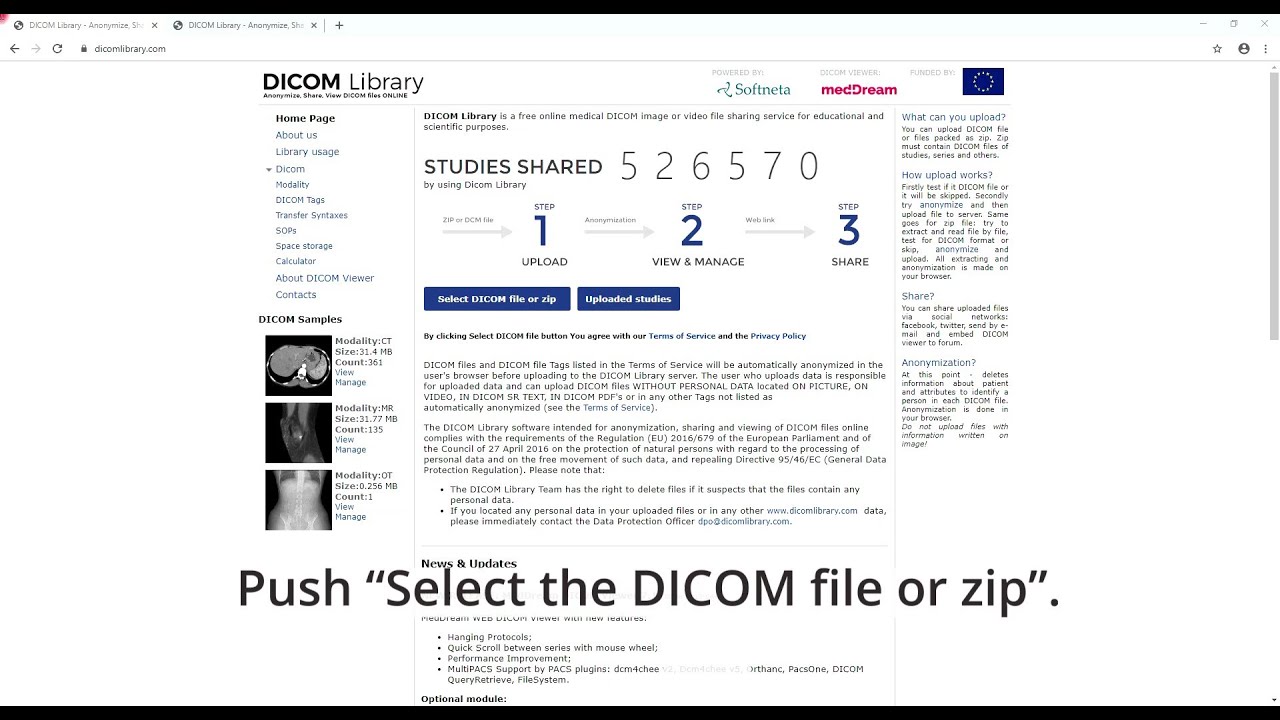A horizontally oriented screenshot captured from a computer screen, likely a desktop or laptop. The image features a thin black border at the top and bottom but not on the sides, indicating it is a full-screen capture.

At the top left, the browser tab reads "DCOM library, anonymize, DCOM library." Adjacent to this are navigation arrows for back and forward, followed by the web address bar. To the top right, there are three window management icons: minimize, maximize (full screen), and close (X). Below this, additional browser controls such as a star for bookmarks, a circular icon, and three vertical dots for more options are visible.

The central portion of the screen showcases a webpage with a clean, white background. At the top, "DCOM library" is prominently displayed, followed by the title "Home Page" in bold. The page features clickable blue links directing the user to various sections.

An article dominates the middle area, introducing the DCOM library as a "free online medical DICOM image or video file sharing service for educational and scientific purposes." It includes statistics on how many times it has been shared and provides further information and samples.

To the left side of the layout, there are sample files or related content listed. At the bottom, users have the option to either select a DICOM file or a zipped file, corresponding with the bottom black border.